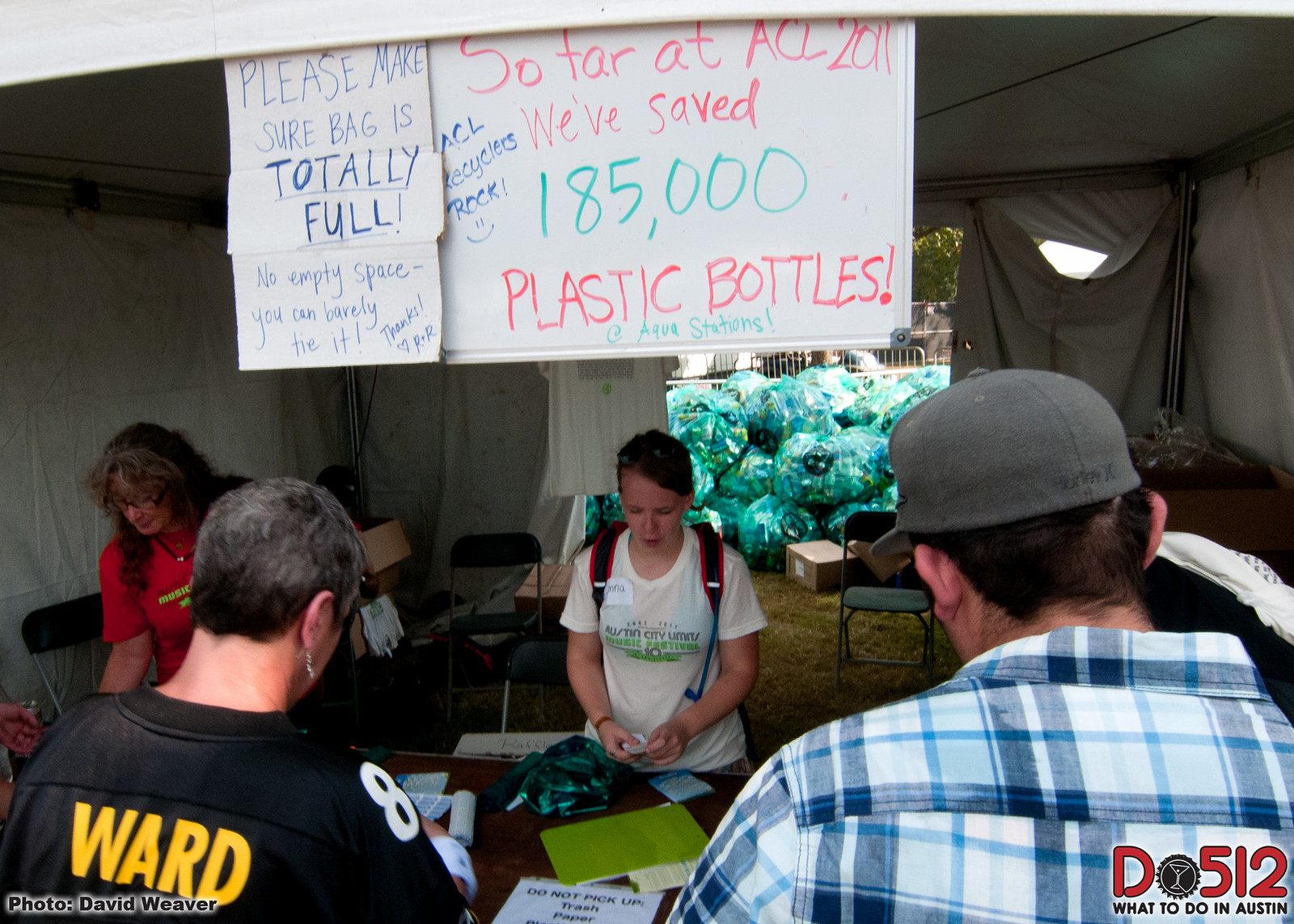This photograph depicts an outdoor recycling event focused on collecting plastic bottles. At the center of the image is a booth resembling a small tent, manned by two individuals—one wearing a black shirt and the other sporting a blue and white checkered shirt—who are assisting two other individuals with their backs to the camera. These two individuals appear to be turning in their plastic bottles at a desk covered in environmental literature.

Above the booth, hanging in clear view, are two white paper signs written in magic marker. The left sign instructs, "Please make sure the bag is totally full. No empty space, you can barely tie it." The right sign proudly proclaims, "So far at ACL 2011 we've saved 185,000 plastic bottles," although additional text is partially obscured and unreadable.

In the background of the scene, numerous green plastic bags filled with bottles are visible, presumably waiting to be processed and recycled. The overall atmosphere suggests a dedicated effort towards environmentalism and community participation in recycling activities.